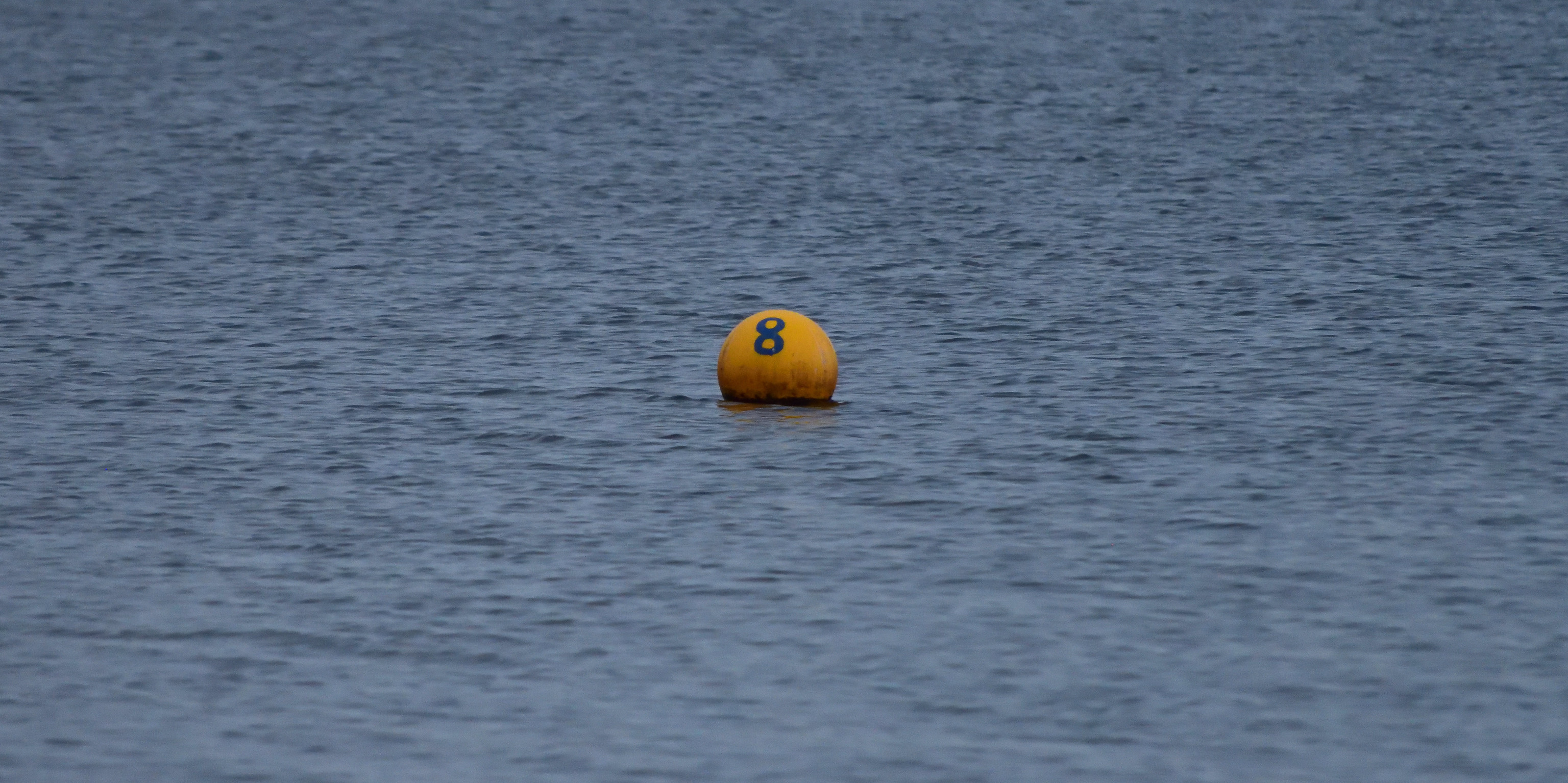The photograph captures a calm, dark blue body of water, likely an ocean. Gentle ripples traverse the surface, giving a sense of subtle movement. Situated in the center of this serene scene is a brightly colored buoy, predominantly orange with an unmistakable number 8 in dark blue or black writing. The buoy is round and ball-shaped, with the bottom quarter submerged, resulting in a darker stain creeping halfway up its surface, indicating its interaction with the water. The overcast sky contributes to the absence of reflections, making the water appear almost a flat hue with no glaring highlights. This singular buoy, partially stained and bobbing gently, stands out vividly against the expansive, rippling blue backdrop.